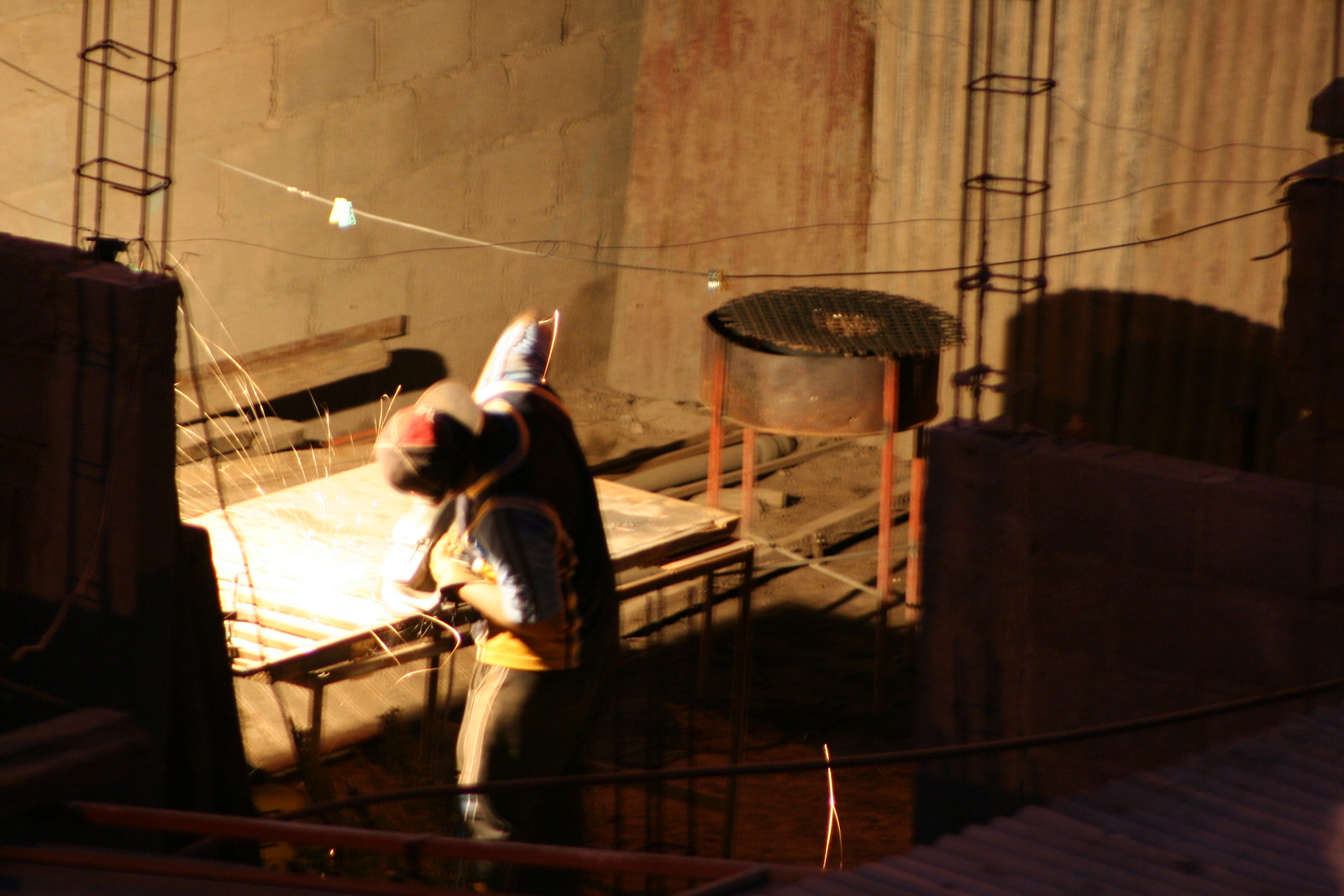The image depicts a welder engrossed in his craft, working diligently on a sheet of metal which produces a cascade of bright sparks illuminating the dimly-lit workspace. The scene is set in an industrial environment, perhaps a warehouse, featuring a backdrop with a stone wall to the left and various metal objects, including a cauldron-like item, scattered in the shadows. The welder, seen from a slightly overhead angle, is attired in a backwards black hat, a basketball jersey revealing short sleeves, and black pants. His hands are protected by gloves, though there's a noticeable gap between the gloves and the sleeves. The welder appears to be in motion, creating a slight blur near his right elbow. The focused light from his welding activity stands in stark contrast to the otherwise shadowy surroundings.